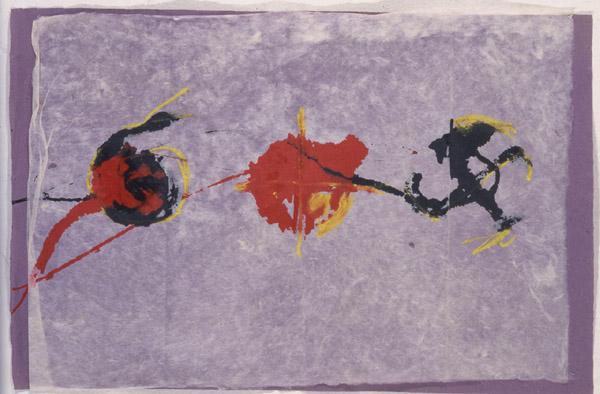This landscape orientation painting, titled "Inner Space 1987" by Luciano Bartolini, is an abstract modern artwork set against a purple background. A wet, white piece of paper overlays the purple backdrop, framed by a white border. The composition features three distinct, abstract forms across the center. On the left, a red and yellow-tinted stem with a flower-like shape is depicted. The middle section showcases a central red blotch with surrounding yellow highlights. To the right, a black, swastika-like shape garnished with yellow accents is visible. The overall palette includes gray, purple, off-white, black, red, and yellow, giving the piece a spectrum of vibrant contrasts and intricate details.